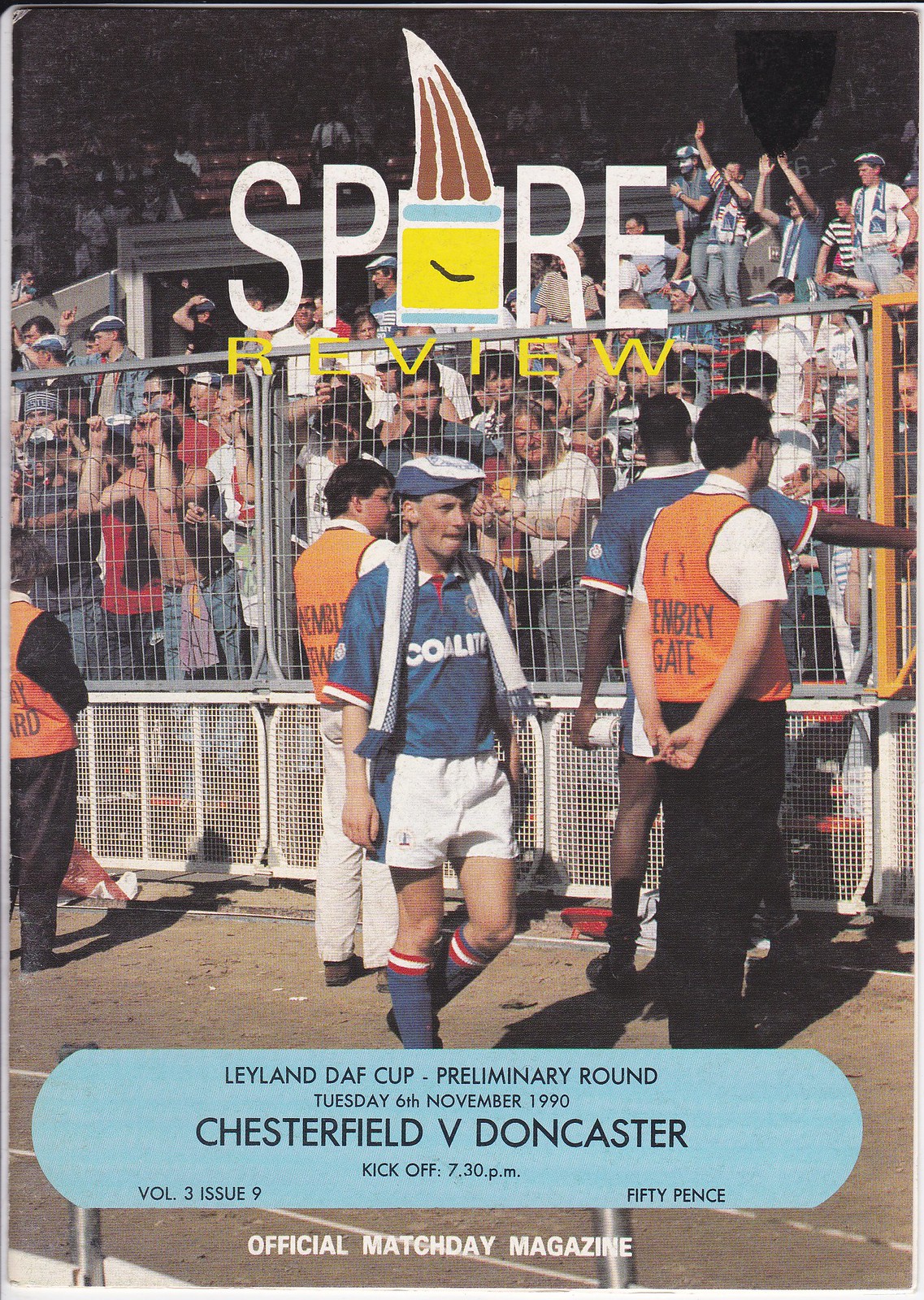This poster for a sports event captures a vibrant scene at a stadium. The background photograph reveals an enthusiastic crowd of spectators in the stands, separated by a metallic fence and boundary. The stands feature multiple ascending rows filled with people, some with their hands raised. Beyond the fence, several employees in orange vests, possibly security guards, can be seen watching the event.

In the foreground, there is a dirt track where a player dressed in a short-sleeved blue athletic outfit with white shorts and tall blue socks is walking. He sports a beret cap, adding a distinctive touch to his appearance.

At the top of the image, the title "Spare Review" is prominently displayed. The event information is located at the bottom, reading: "Leyland Deaf Cup preliminary round, Tuesday, 6th November 1990, Chesterfield versus Doncaster, kick-off at 7.30 p.m., Volume 3, Issue 9, 50 pence, official matchday magazine." This detailed text provides specific details about the sports event, enhancing the overall significance of the poster.